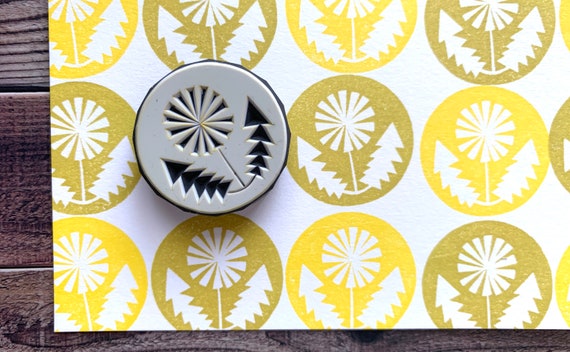This image features a light gray cylindrical stamp, likely used for creating decorative patterns. The stamp's design depicts a central circular flower with a tiny center and spiked petals, flanked by two curved branches resembling pine trees at its base. Each branch consists of five small triangles in a row. This item rests on a piece of white paper, which has been repeatedly stamped with the same intricate image in alternating shades of yellow and yellow-green ink. This stamped paper lies on a dark wooden table, providing a rich, contrasting backdrop. The overall impression is one of an intricate, nature-inspired pattern possibly intended for use as a decorative element or on gift wrap.